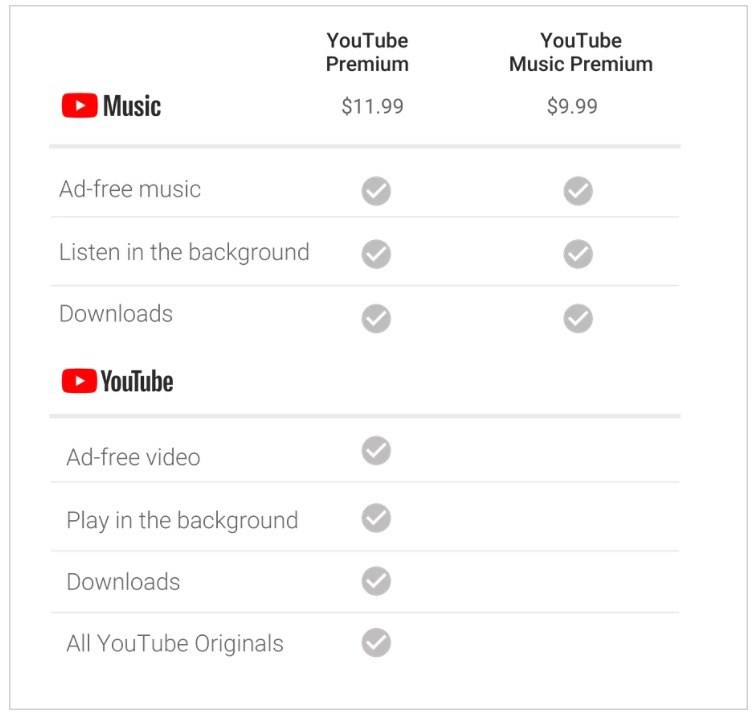The infographic presents a comparison between YouTube Premium and YouTube Music Premium on a clean, white background divided into two columns. The left column represents YouTube Premium, while the right column represents YouTube Music Premium.

At the top of the infographic, both columns feature the familiar YouTube play icon - a red rectangle with a white play button. Next to this, the text "Music" is displayed to indicate the different services. The pricing is listed beneath the icons, with YouTube Premium priced at $11.99 per month and YouTube Music Premium at $9.99 per month.

The benefits of both services are illustrated using gray circles containing white check marks. Under both columns, it is indicated that both YouTube Premium and YouTube Music Premium offer ad-free music, the ability to listen in the background, and music downloads.

Further down the infographic, additional benefits exclusive to YouTube Premium are listed, again marked by gray circles with white check marks in the YouTube Premium column only. These benefits include ad-free video, background playback for all video content, video downloads, and access to all YouTube Originals.

The graphic provides a clear, side-by-side comparison, helping users easily differentiate between the two subscription services and their respective features.